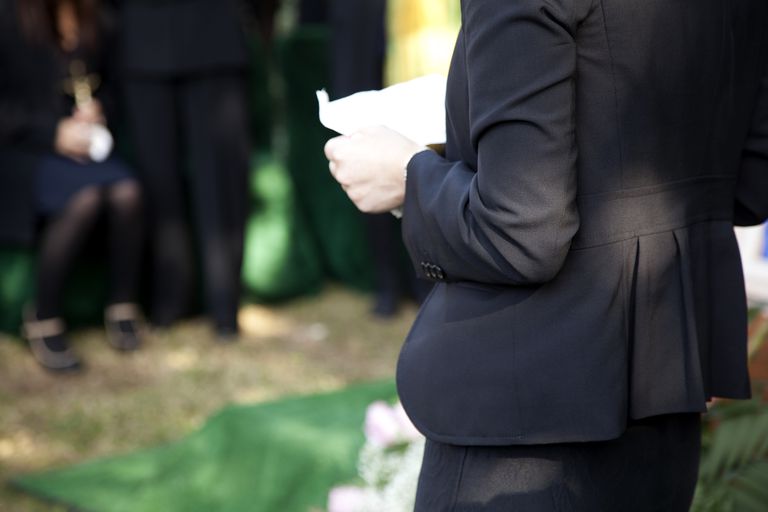The image captures a solemn outdoor scene, likely at a funeral. Dominating the foreground on the right side is the back of a person dressed in a dark suit. Their head, neck, and shoulders are out of frame, but their posture is clear—arms bent at 90 degrees, with hands positioned in front of their abdomen holding a white piece of paper, their left fist partially visible. The camera focuses on the person's black jacket and pants while blurring the background. In the background, other figures dressed in dark attire can be seen standing and sitting, their forms indistinct. The group is positioned on a grassy area, with a more pronounced green swath on the ground, potentially suggesting a floral arrangement. Soft rays of light filter through, adding a serene touch to this mournful gathering.